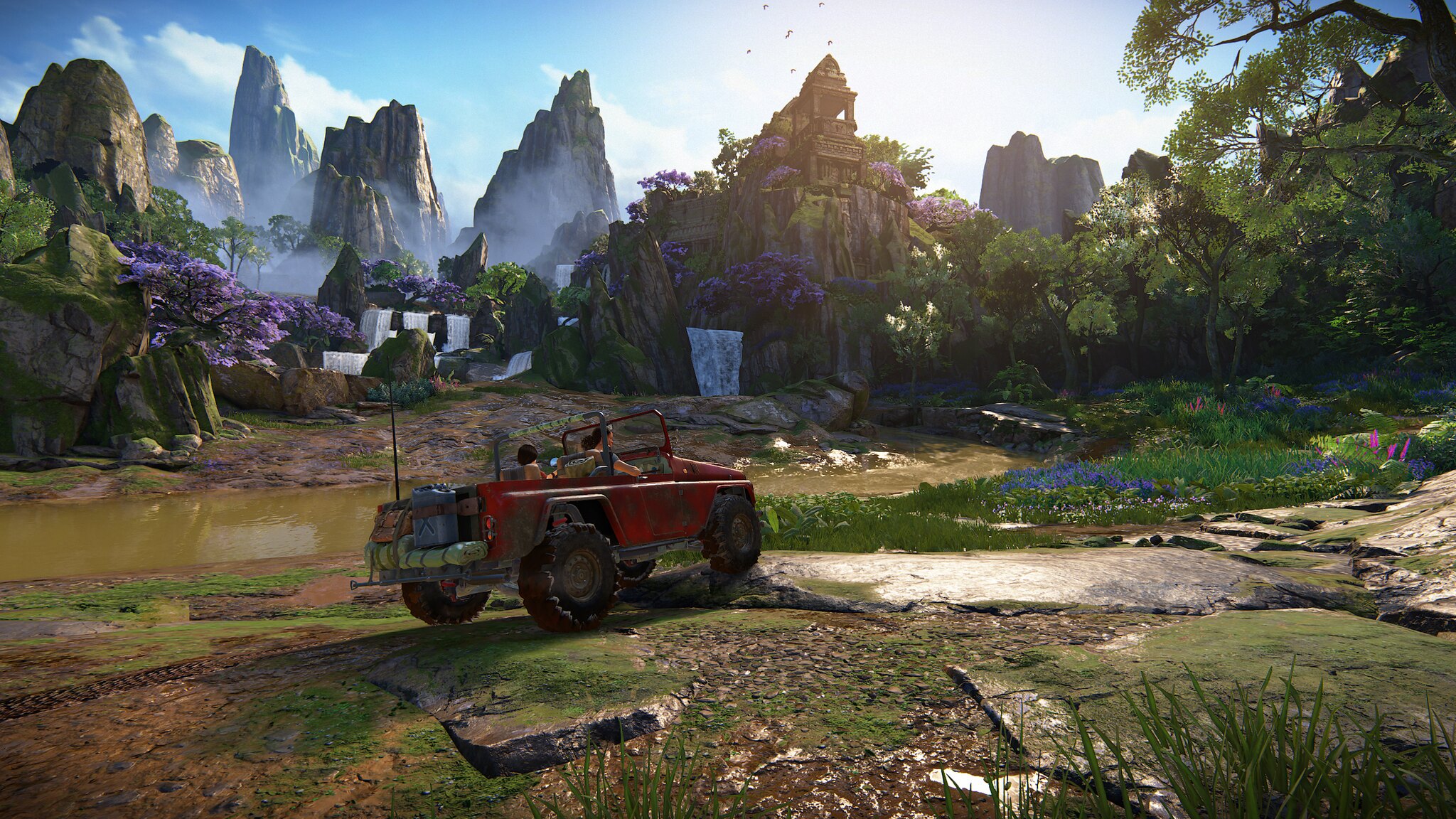In this captivating screenshot likely taken from a video game, a vibrant red Jeep without a top is prominently featured. Inside the Jeep, two characters are visibly seated, and we observe the vehicle from a rear, 45-degree angle as it navigates a muddy, stone-covered path. The backdrop is a breathtaking, striking landscape adorned with cascading waterfalls and towering mountains. Beautifully contrasting with the rugged terrain are trees adorned with ethereal purple flowers. In the distance, an idyllic meadow blooms with various flowers, contributing to the picturesque scenery. Atop one of the majestic mountains, the remnants of an ancient-looking structure, possibly a temple, are faintly discernible, adding an element of mystery and historical intrigue to the scene.